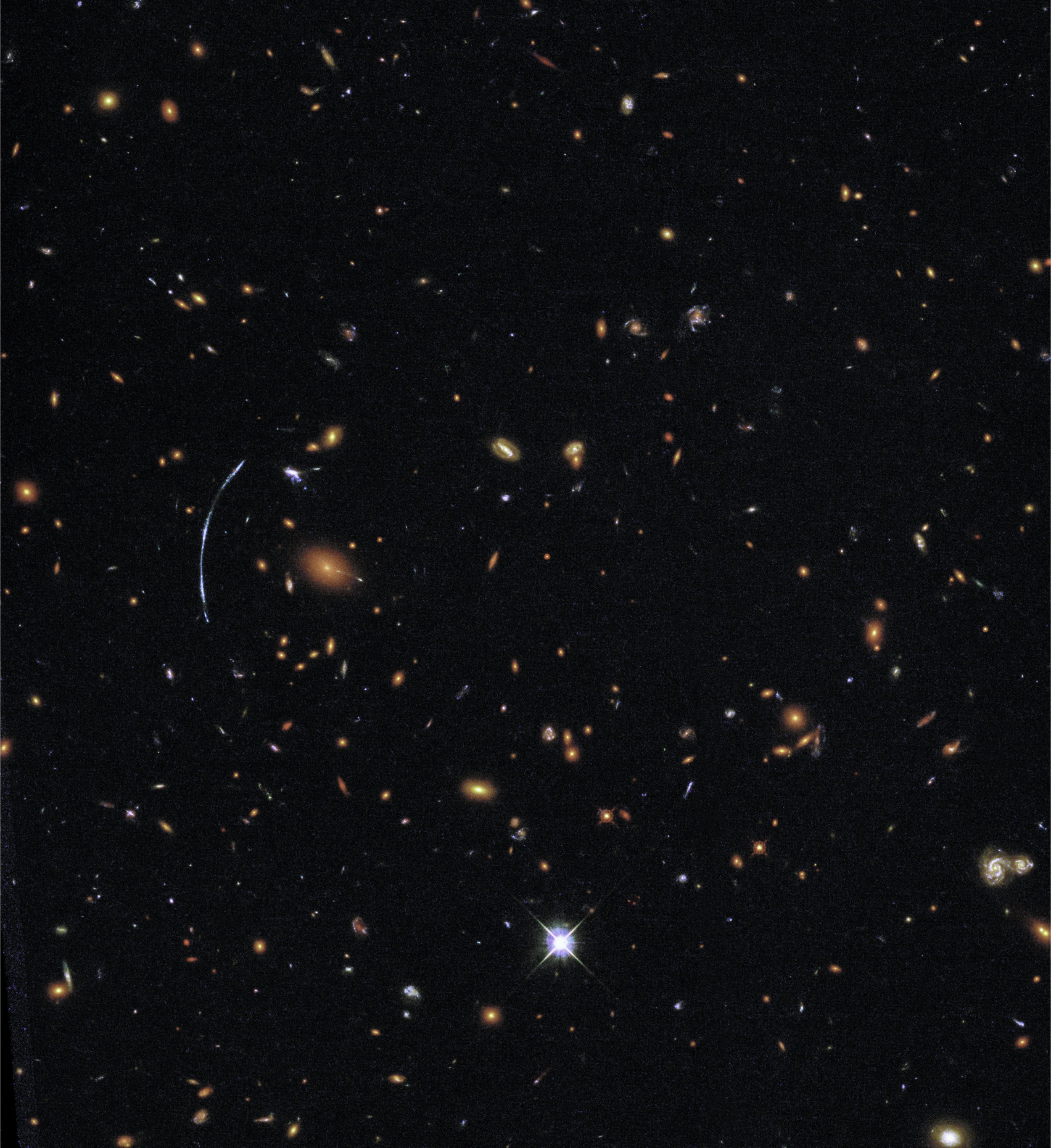This stunning, digitally captured image of deep space, presumably taken by a powerful telescope such as the Hubble Space Telescope, features an incredibly black background that emphasizes the celestial tapestry within it. Scattered across this dark expanse are numerous glowing points of light in varying hues—bright whites, warm yellows, vibrant oranges, subtle blues, and occasional browns—representing stars, galaxies, and perhaps even nebulae. Toward the bottom center, a radiant white star stands out, distinguished by a prominent four-pointed lens flare effect. Amidst the myriad of celestial bodies, several spiral and oval-shaped galaxies can be discerned, providing a sense of the vast depths and complexities of space. There's also a curious white, curved arc shape near the center-left, adding to the enigmatic beauty of the scene. While the exact nature of some objects remains ambiguous, the image presents a breathtaking and awe-inspiring glimpse into the far reaches of the universe.